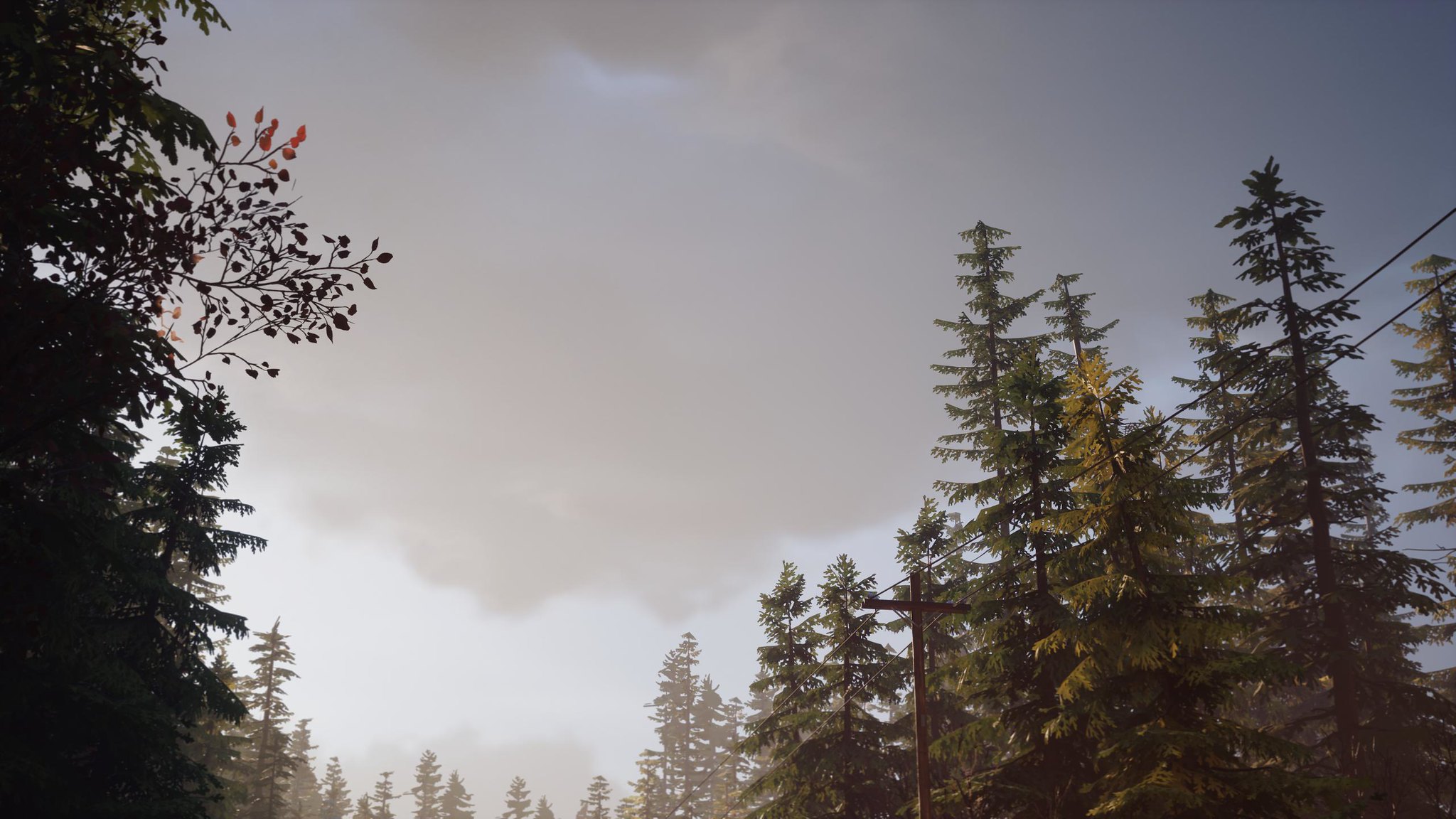The image depicts a dramatic scene in a northern wilderness, likely resembling Alaska, featuring towering spruce trees. The perspective is from the ground looking upward, emphasizing the immense height of the trees, which are predominantly found on the right side and appear to dwarf a visible telephone pole with power lines. In contrast to the robust spruce, more delicate branches with leaves can be noticed on the left side of the photo. The sky above is a mix of moody gray clouds and patches of blue, suggesting an impending storm or heavy cloud cover that casts a dusky light across the scene. The background, which stretches toward the bottom of the image, showcases the distant tree tops, giving a sense of depth and distance. There's also a faint hint of a lighter area in the sky, possibly hinting at the sun trying to break through the cloud cover, adding to the dramatic atmosphere of the photograph.